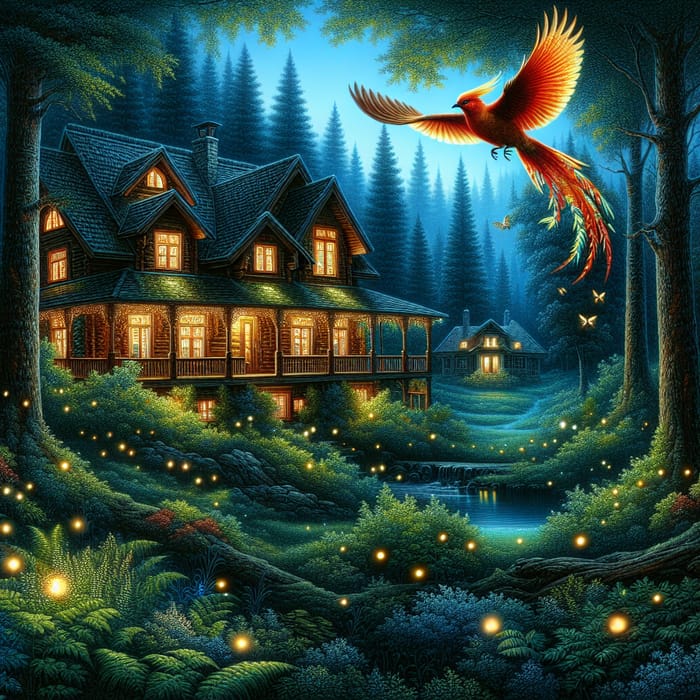This captivating, AI-generated image showcases a vibrant and stylized fantasy setting of a two-story cottage nestled deep within a dense, glowing forest. The main house, possibly a bed and breakfast inn, features a charming wraparound porch and numerous illuminated windows, including an attic window under the arched roof. The scene is set at dusk, with a deep blue hue enveloping the entire landscape, enhancing the magical atmosphere.

In front of the cottage, lush, green foliage comprising various plants and trees surrounds a small body of water, perhaps a pond or stream with a waterfall. The forest extends further into the background, where another smaller and equally illuminated cottage sits, hinting at a possible complex or connected dwelling.

A striking bird, reminiscent of a phoenix, dominates the scene with its vibrant red plumage, yellow crested feathers, and enormous wingspan. It is in mid-flight and accompanied by a flurry of butterflies and fireflies, whose glow adds to the enchanting ambiance. The tall trunks of evergreen trees frame the image, completing this ethereal forest sanctuary.